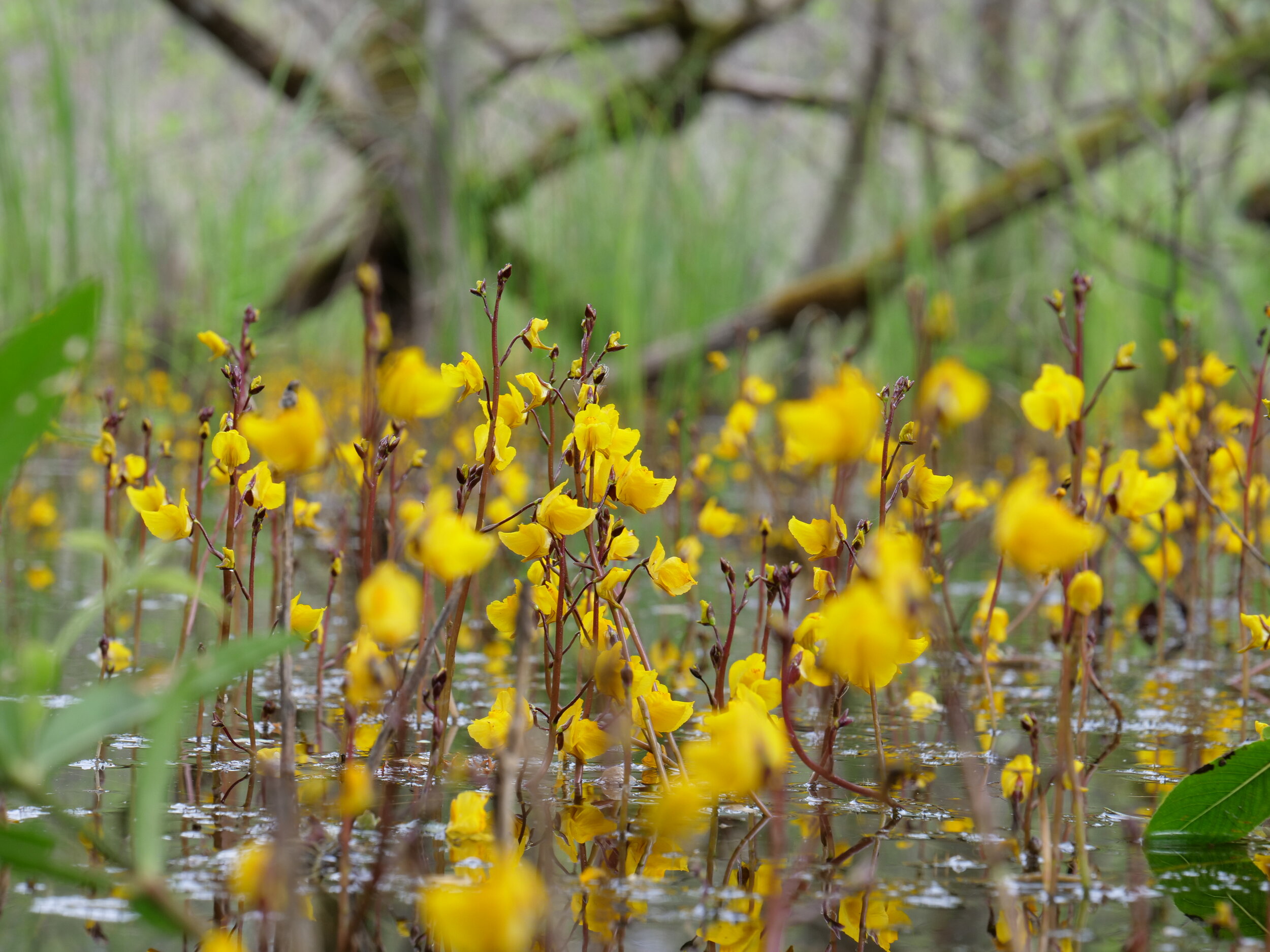The photograph captures a vibrant, sunlit marshland scene during the daytime. The rectangular image, approximately five to six inches wide and four inches high, showcases a pond area in the foreground. Tall, thin reddish-brown stems rise from the water, adorned with numerous small, vibrant yellow flowers and buds. The yellow flowers at the lower part of the image are blurred, while those in the center are sharply in focus, highlighting their delicate beauty. The water beneath the stems appears muddy brown with shimmering silver ripples.

On the lower left, long, narrow leaves attached to a green stem stretch toward the water, contrasting with a wider, elliptical leaf on the lower right, which dips into the pond. The photograph's upper half is blurred, revealing tall green grasses and intertwined dark brown branches in the background. A suggestion of a giant tree that resembles an oak looms further back, though it remains out of focus. The overall scene, possibly reminiscent of an Everglades environment, is rich with green marsh grasses and a mix of tree branches and leaves, capturing the serene beauty of a thriving wetland ecosystem.